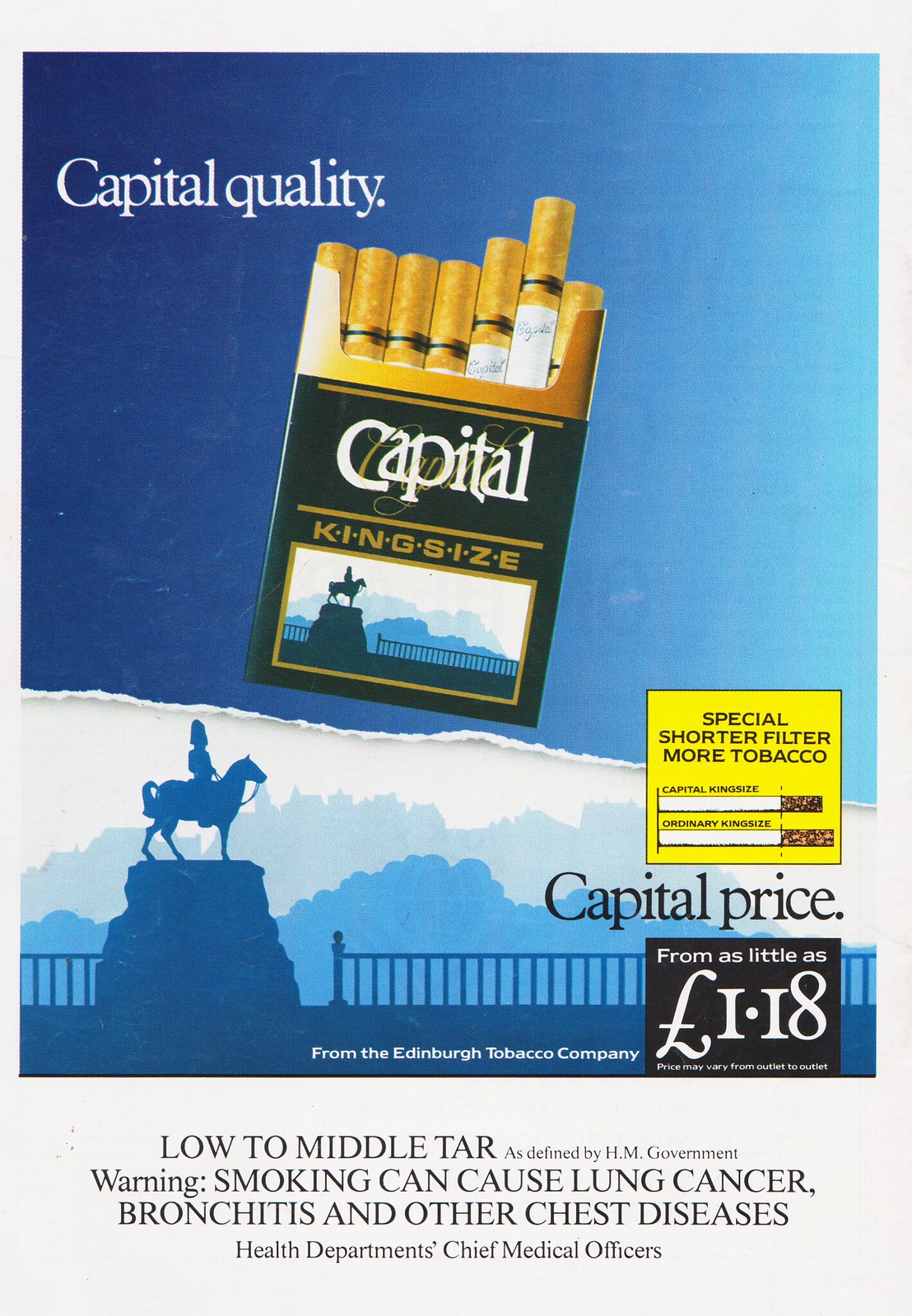This full-page advertisement for cigarettes features a striking design with a gradient blue background, transitioning from dark blue on the left to light blue on the right. Dominating the top portion is a bold white text proclaiming "Capital Quality." Central to the ad is a colored illustration of a dark green and bronze cigarette packet, positioned diagonally. The packaging displays "Capital" in white text and "King Size" in bronze below it. Several cigarettes emerge from the top of the pack.

On the lower part of the packaging, there is an image of a statue depicting a man on a horse, further emphasized by the same historical imagery repeated across the bottom section of the advertisement. Accompanying this visual, a yellow box on the right promotes the product's "Special Shorter Filter for More Tobacco," alongside a comparative drawing of two cigarettes, labeled "Capital King Size" and "Ordinary King Size."

A black square at the bottom advertises the "Capital Price" starting from as little as 1.18 pounds, with the statement "from the Edinburgh Tobacco Company" written in white text. Near the bottom edge, warnings are clearly stated in black text on a white background: "Low to Middle Tar, as defined by HM Government. Warning, smoking can cause lung cancer, bronchitis, and other chest diseases." alongside the endorsement from the "Health Departments, Chief Medical Officers."